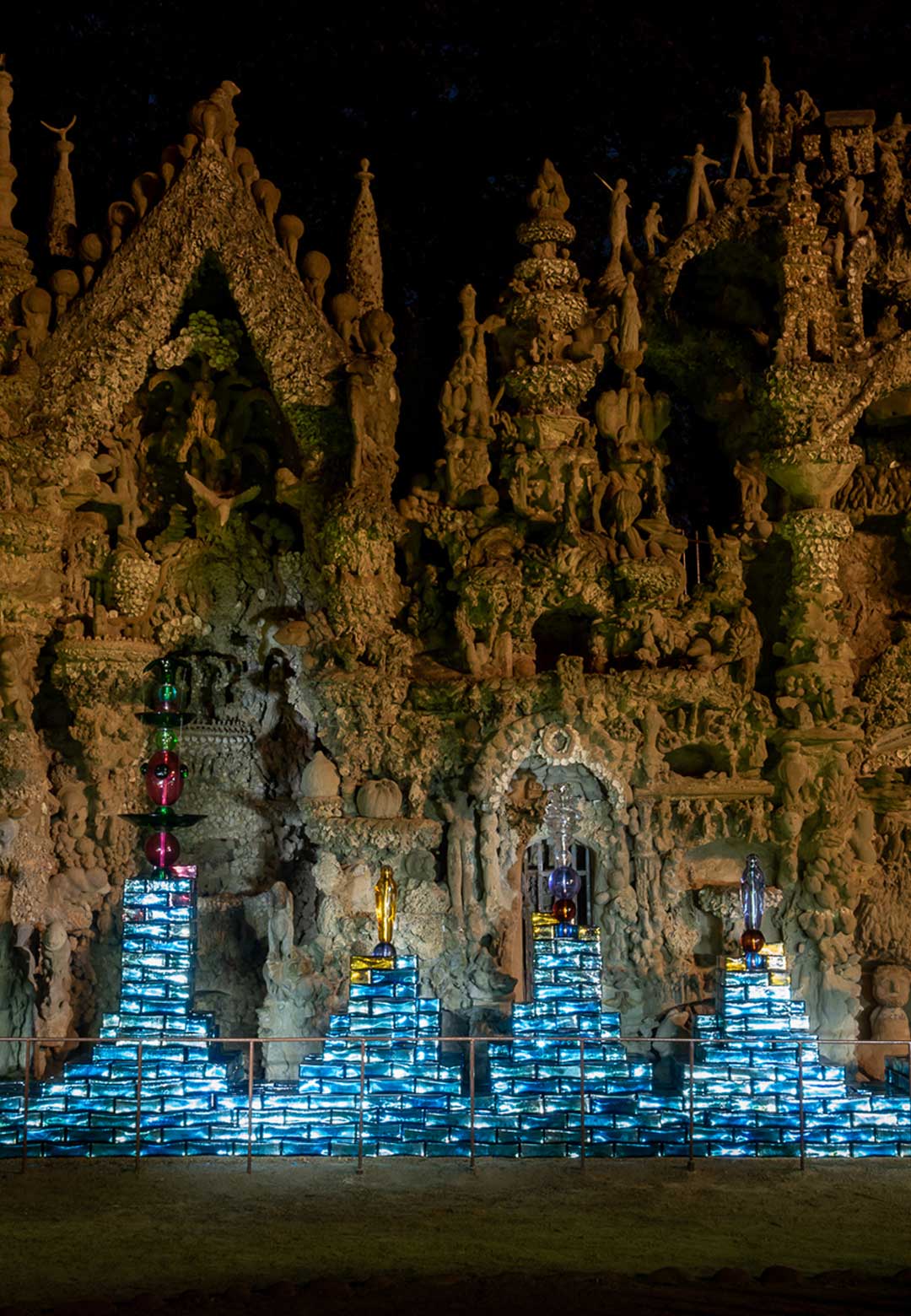This nighttime photo captures a stunning scene featuring what appears to be an ancient city that mimics intricate Hindu design. Dominating the background is a highly ornate structure, evocative of a palace or temple, characterized by intricate stone carvings and conical spires made from rock, possibly carved from a mountain or hill. The structure includes delicate figures of people and animals, further emphasizing its meticulous craftsmanship.

In front of this grand monument, there are modern sculptures comprising columns of blue blocks that resemble glass bars stacked vertically. Each column supports unique, illuminated glass vases that add a touch of contemporary art to the historic backdrop. These glass structures are multi-colored, showcasing shades of gold, purple, green, pink, and black, and their patterns and illuminations create captivating reflections and shadows on the ancient structure behind.

The entire scene is enclosed by a fence, adding a layer of separation between the artifacts and the dark green ground beneath, which is faintly visible. The juxtaposition of ancient and modern elements, all bathed in light, crafts a mesmerizing tableau that is both timeless and contemporarily vibrant.